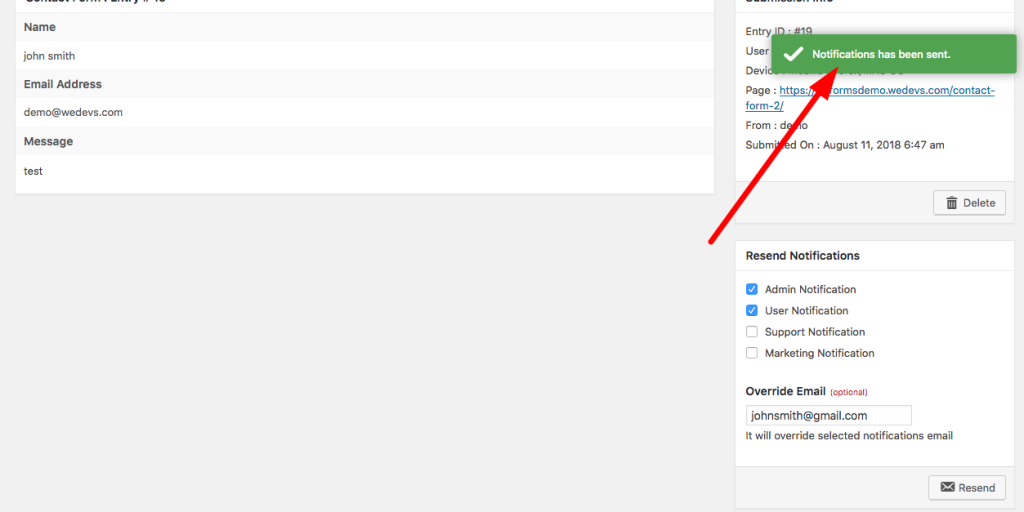The image appears to display a user interface, which could either be a website or an app, as the address bar is cropped out. In the top right corner, there is a striking green rectangular pop-up box featuring a white check mark and a message indicating that notifications have been sent. A red arrow, photoshopped into the image, points directly at this notification.

In the main section of the interface, set against a gray background, there is detailed user information. On the upper left, we see: 
- **Name:** John Smith
- **E-mail address:** demo@WEDEVS.com
- **Message:** test

To the right, partially obscured by the pop-up, are additional details:
- **Entry ID:** 19
- **Source:** demo
- **Submission Date and Time:** August 11th, 2018 at 6:47 AM

In the bottom right of this section, there's a delete button for removing the entry. Below this, options for re-sending notifications are displayed. Check marks indicate that:
- **Admin notification** and **User notification** have been selected for re-send.
- **Support notification** and **Marketing notification** are not selected.

There is also an optional override email field: johnsmith@gmail.com, which, if filled, will replace the selected notification emails. A re-send button is available in the bottom right corner to apply these changes.